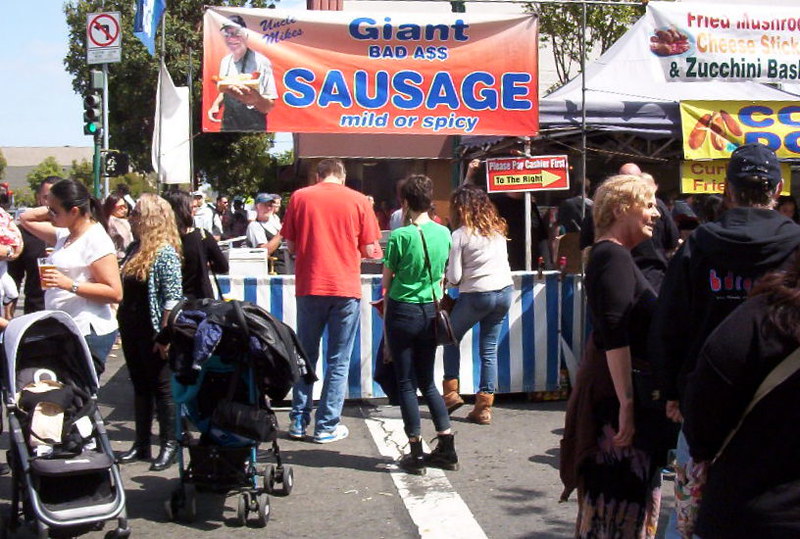The photo captures a bustling farmer’s market or fair, teeming with people and energy. Central to the scene is a busy food booth with a striking banner that reads "Giant Bad Ass Sausage" in blue text on an orange background, offering both mild and spicy sausages. The banner also features an image of a smiling man holding a sausage in a bun, labeled "Uncle Mike." At the booth, a blue and white striped flag drapes below the counter, and a sign directs customers to pay the cashier first. In front of the booth, the backs of three people—a woman in white, another in green holding a purse, and a man in an orange shirt—are visible as they wait for their orders. Adjacent to this, a white-topped tent with a yellow banner advertises "Fried Mushrooms, Cheese Sticks, and Zucchini Baskets," along with images of the food and the beginnings of a sign for "Curly Fries." Patrons with drinks engage in conversation while others navigate the crowd with baby carriages. Trees and streetlights dot the background, contributing to the lively fair atmosphere.